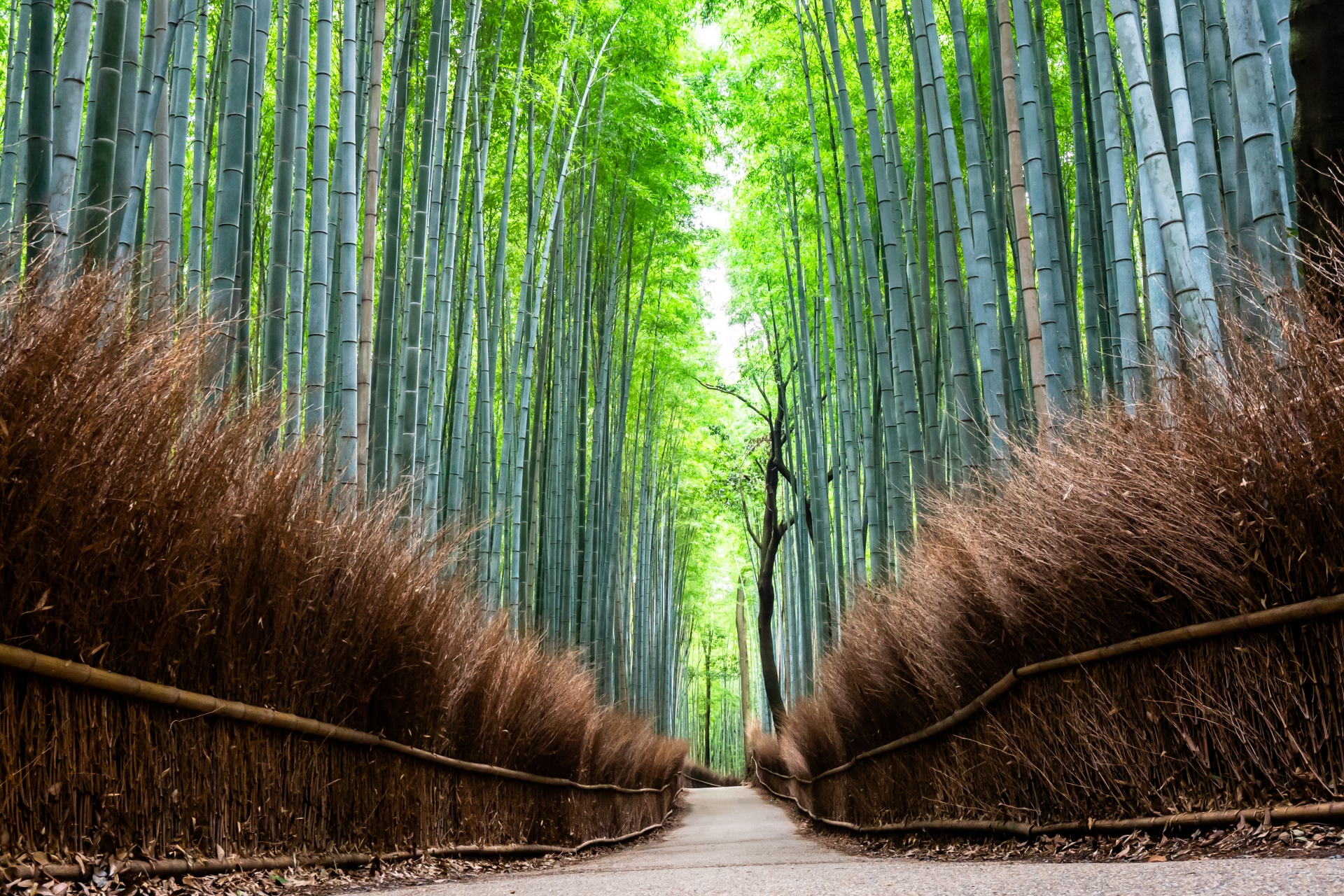The image showcases a narrow cement walkway, cutting through a dense, modified forest area. The walkway is surrounded by a striking arrangement of tall, thin tree trunks or bamboo, soaring up and creating an arch-like effect that envelops the path, making it feel like a natural tunnel. Flanking the path on both sides are long, straw-like brown bushes, contained within dark brown or bamboo-like borders. The bushes stretch along the entire length of the trail, contributing to its secluded, enclosed atmosphere. Above, the rich greenery of the tree or bamboo leaves contrasts with the brown of the bushes below and creates a canopy that allows sunlight to filter through. The scene is reminiscent of a church archway, creating a serene and enchanting passage through the forest.